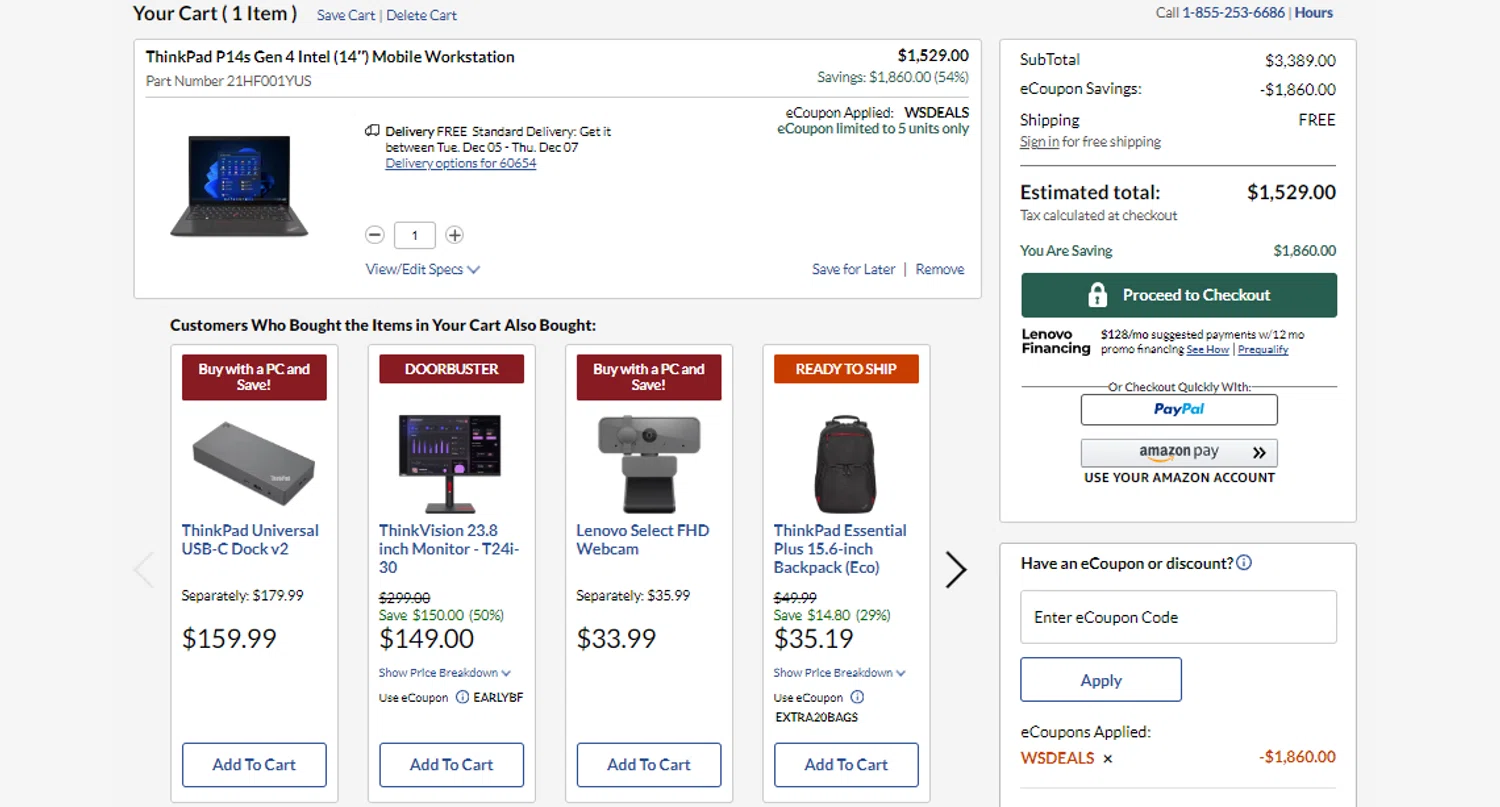This image depicts a detailed overview of an online store's shopping cart page. The primary item in the cart is a "ThinkPad P14s Gen 4 Intel," described as a 14-inch mobile workstation. Beside it, various interactive options such as "Save Cart" and "Delete Cart" are visible. The part number specific to this ThinkPad model is also listed, accompanied by an icon representing the laptop.

Highlighted details include free standard delivery, with a specified delivery range between Tuesday, December 5, and Thursday, December 7. The listed price for the laptop is $1,529, reflecting a significant saving of $1,860 due to an applied e-coupon, which is limited to five units. 

Below this listing, there is a section suggesting additional items typically purchased by other customers who bought the same laptop. Recommendations include:
1. ThinkPad Universal USB for $159
2. ThinkVision 23.8-inch Monitor for $140
3. Lenovo Selective FHD Webcam for $33.99
4. ThinkPad Essential Plus 15.6-inch Backpack for $35

On the right side of the page, financial details of the shopping cart are summarized, including the subtotal, e-coupon savings, shipping charges, and the estimated total, ensuring a transparent shopping experience.